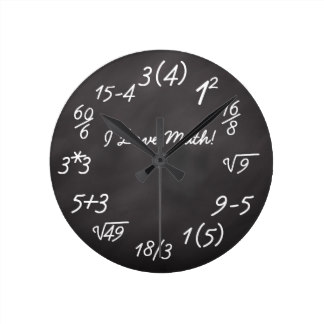This is a computer-generated image of a distinctive wall clock with a minimalist black and white design, set against a transparent white background. The clock features a black round base reminiscent of a chalkboard, and its black hour, minute, and second hands point to a unique sequence of mathematical expressions instead of traditional numerals. Each hour position is represented by a formula: 
- 12 o'clock is denoted by "3(4)"
- 1 o'clock by "1 squared"
- 2 o'clock by "16 divided by 8"
- 3 o'clock by "the square root of 9"
- 4 o'clock by "9 minus 5"
- 5 o'clock by "1(5)"
- 6 o'clock by "18 divided by 3"
- 7 o'clock by "the square root of 49"
- 8 o'clock by "5 plus 3"
- 9 o'clock by "3*3"
- 10 o'clock by "60 divided by 6"
- 11 o'clock by "15 divided by 4"

In the clock's center, written in cursive, is the phrase "I love math!" with an exclamation point. The time displayed is 10:10, with the second hand at 6, a common configuration for promotional clock images.